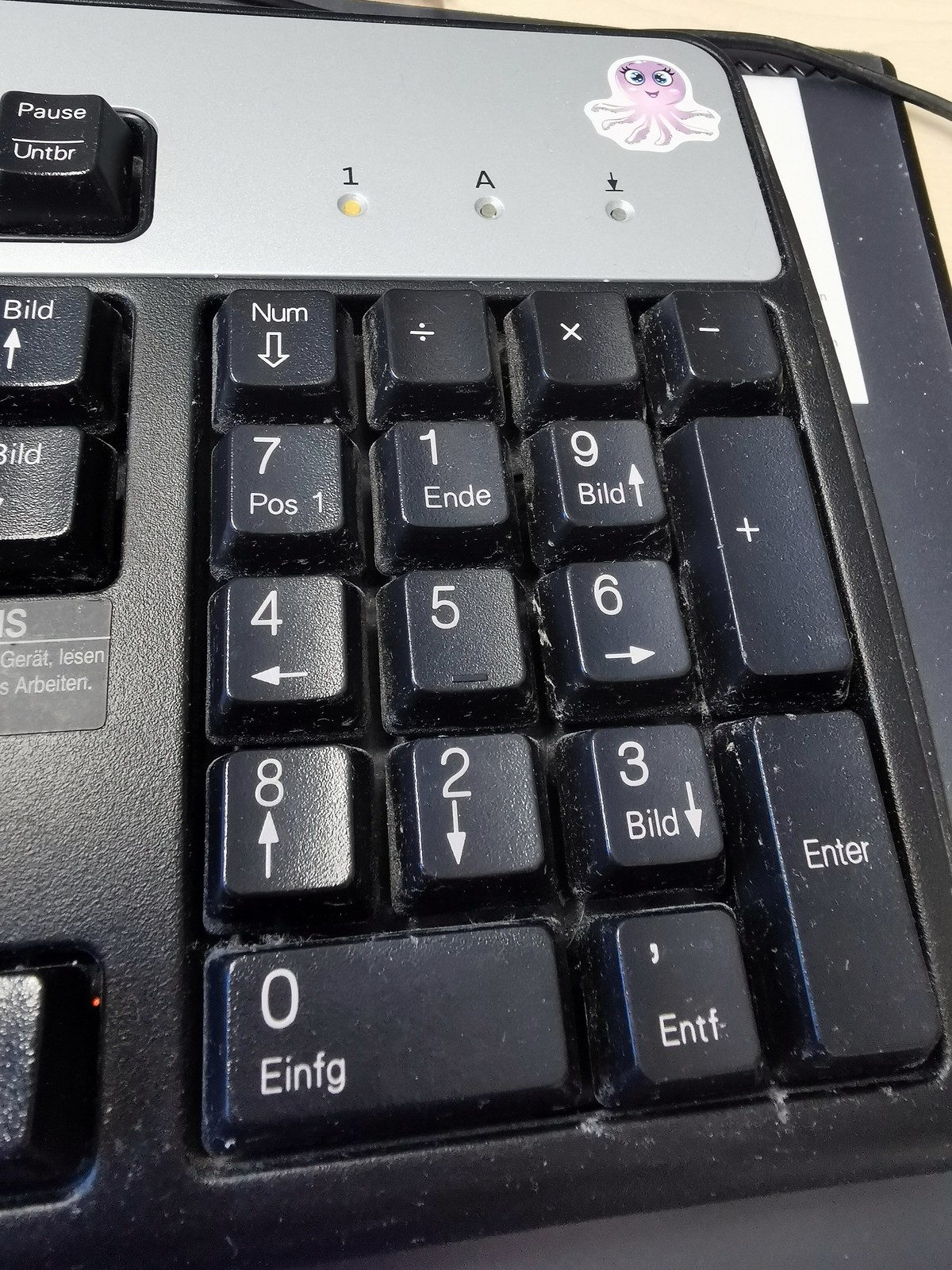This image depicts a detailed portion of a dusty and grime-covered black keyboard, which appears to be configured in a non-standard layout and possibly in a foreign language. The keyboard features both English words and what seems to be another language, possibly German. 

In the numeric keypad section, which is in the alpha-numeric pad layout, the numbers are oddly arranged from top to bottom and left to right: 7, 1, 9, 4, 5, 6, 8, 2, 3, suggesting keys like 1 and 8 might be switched, with the arrow on the 8 key improperly pointing upwards. A light indicator, under the number 1, shows that a specific lock feature is activated. Adjacent to this lit-up section is a key labeled "PAUSE" with a translated equivalent in the other language beneath it.

At the top right corner, the keyboard has a distinctive pink octopus sticker with blue eyes, a smiley face, and white-tipped tentacles. This octopus also has eyelashes, giving it a feminine appearance. Behind the keyboard, a piece of white paper is partially visible. Notably, a black cord extends out from the same upper corner.

In the center, part of a black label with text in a foreign language is visible, further indicating the non-English nature of this keyboard. The entire keyboard is set against a silver backdrop along the top edge where the light indicators for Num Lock and Caps Lock are situated. The pervasive dust and small white specks scattered near the keys further underscore the neglected and dirty state of the keyboard.